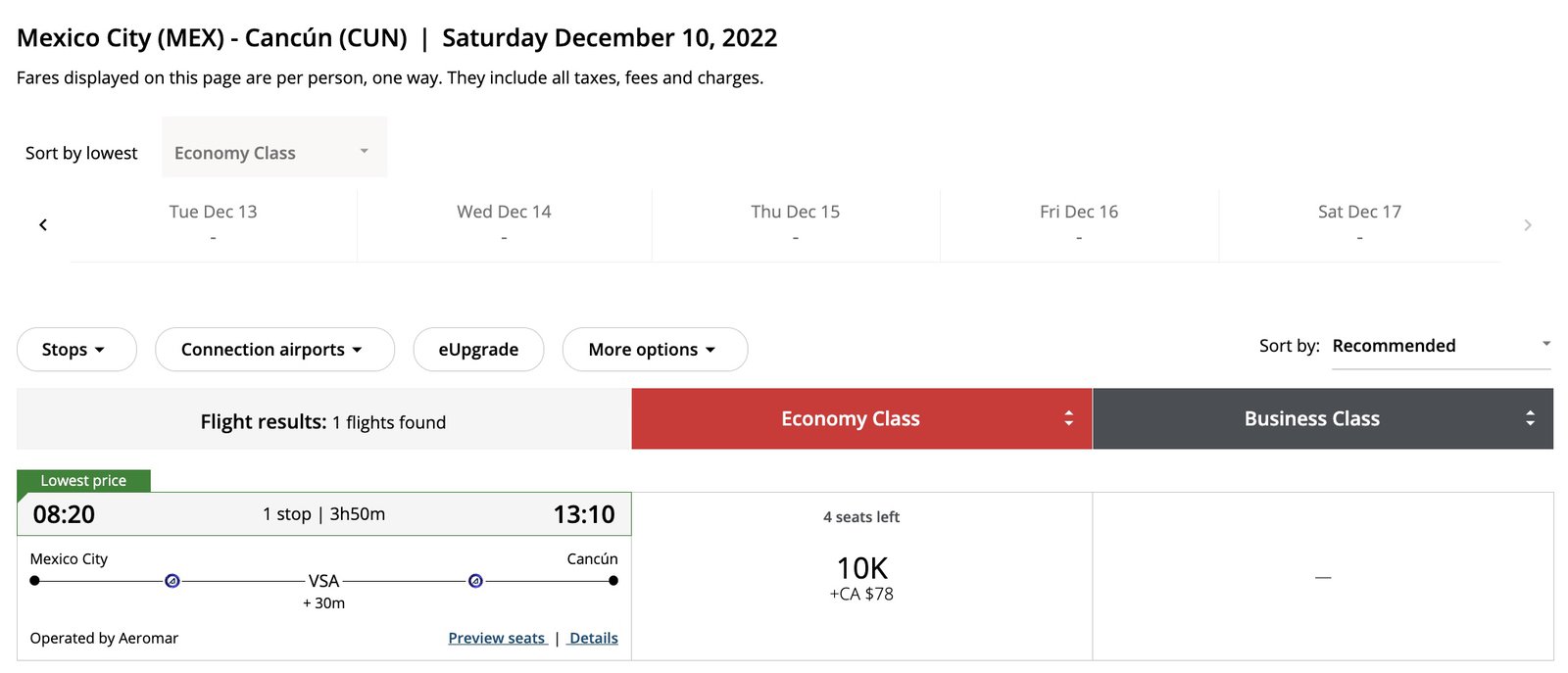Screenshot of a travel booking webpage for a trip from Mexico City (MEX) to Cancun (CUN) on Saturday, December 10th, 2022. The page displays all fares per person for one-way trips, inclusive of all taxes, fees, and charges. 

At the top, there are sorting options. A `Sort by lowest` button is selected on the left side, next to a grayed-out button indicating additional sorting choices. The sorting is currently set to economy class. 

Below the sorting options, a range of selectable dates spans from Tuesday, December 13th to Saturday, December 17th, abbreviated as TUE, WED, THU, FRI, and SAT. 

In the center of the page, there are buttons for filtering by stops, connecting airports, economy upgrade (E-upgrade), and more options. Towards the right, another `Sort by` button is displayed, set to `recommend`.

Further down, the search results show one available flight: 

- Departs at 08:20 (820 Hours)
- One stop with a total flight duration of 3 hours and 50 minutes (3H50M)
- Arrives at 13:10

Flight details: Mexico City to Cancun, operated by Aromar. A button is available to preview seats and details.

At the bottom, there are options indicating seat availability and fare classes:
- Economy class: 4 seats left, priced at 10,000 pesos (10K)
- Business class: options not detailed in the provided text but indicated with colored boxes (red for economy, black for business).